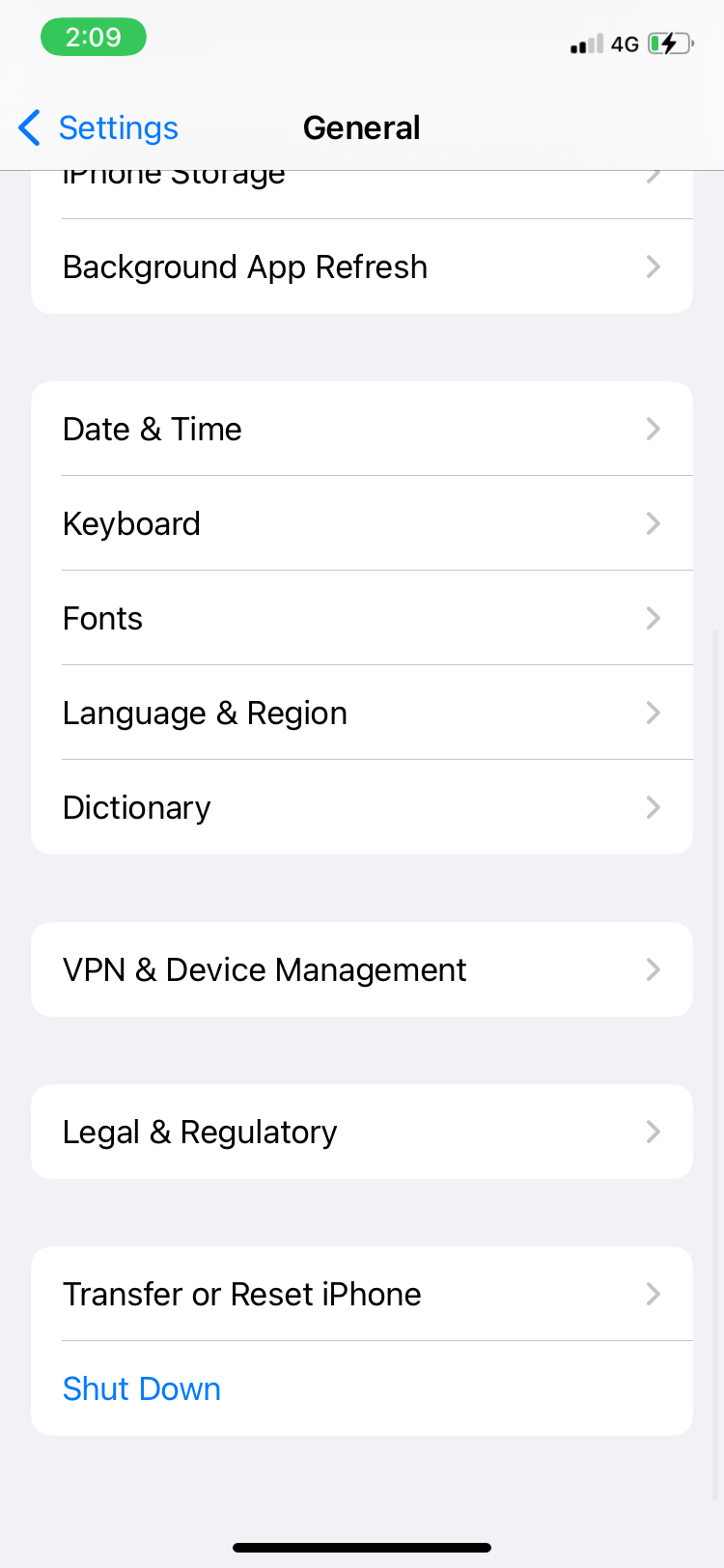The image depicts the screen of an iPhone with the "Settings" app open to the "General" settings section. At the very top left corner of the screen, there is a green circle displaying the time "2:09." To the right of the time are four signal bars, with the first two bars filled in black, indicating signal strength. Further to the right, it shows "4G" connectivity and a battery icon that is nearly depleted, with only a small amount of green remaining. 

Below the status bar, a gray heading section has the word "Settings" in blue on the left and "General" in black towards the right. Underneath this heading, the screen is divided into two prominent sections. The first section presents options labeled "iPhone Storage" and "Background App Refresh," each within a separate gray-bordered rectangle.

Continuing down, there is another larger white rectangle divided into five subsections, each bordered in gray. These subsections are labeled sequentially as "Date & Time," "Keyboard," "Fonts," "Language & Region," and "Dictionary."

Further down, separated by a gray border, the headings "VPN & Device Management" and "Legal & Regulatory" are listed, each followed by a gray border. Lastly, there is a final white rectangle divided into two options: "Transfer or Reset iPhone" and a blue-colored "Shutdown" link. At the bottom, there is a gray border with a black horizontal line running through the middle.